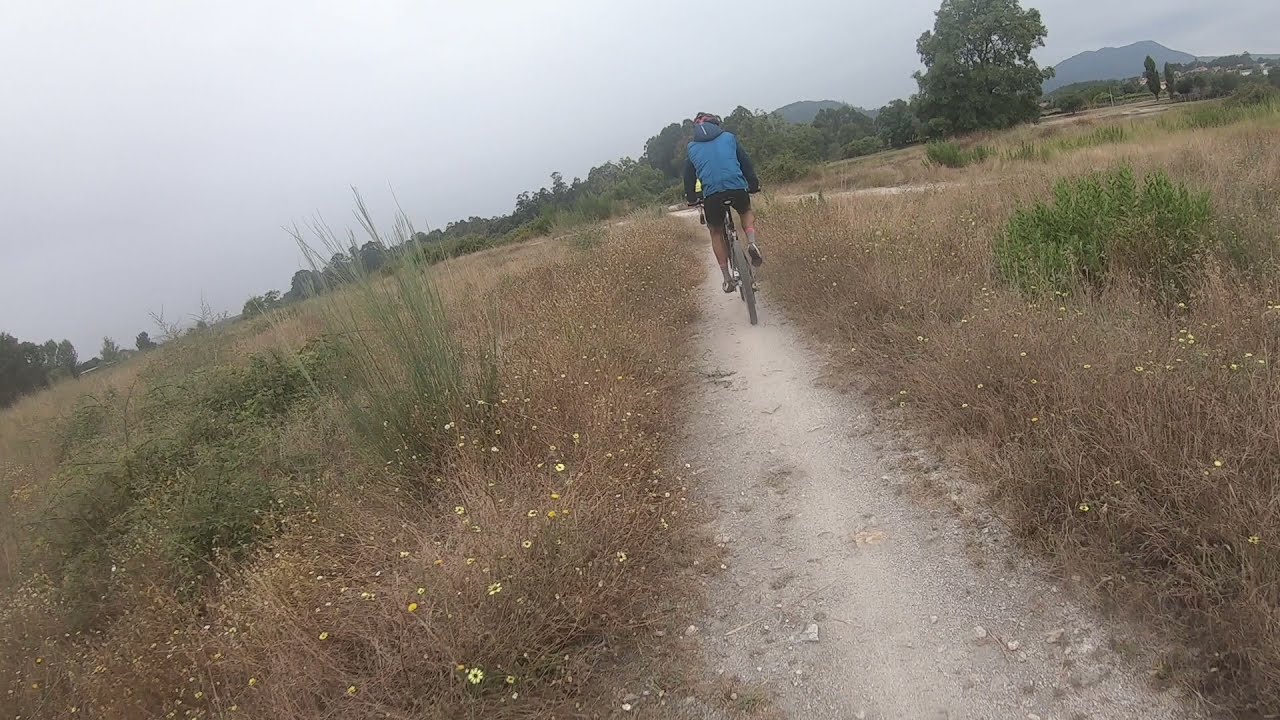The image depicts a remote, unpaved dirt path bending slightly to the left. A bicyclist, wearing black shorts, a blue jacket with black sleeves—a hoodie to shield from the overcast gray skies—is riding away from the camera. His bike, a dusty gray, and his left leg is extended downward, just touching the ground while his right leg is slightly raised. Dense grayish and green weeds flank the trail, emphasizing its rugged nature. The path, sparsely vegetated with small green bushes and dry brush, weaves through a landscape dotted with larger bushes and a few sizable trees. In the top right corner, the silhouette of rocky mountains looms in the distance under the cloudy sky, hinting at an impending rain shower. Further to the right, the faint outline of a suburban dwelling peeks from behind the greenery. The solitary rider is the sole occupant of this scene, adding to the tranquility of the natural setting.